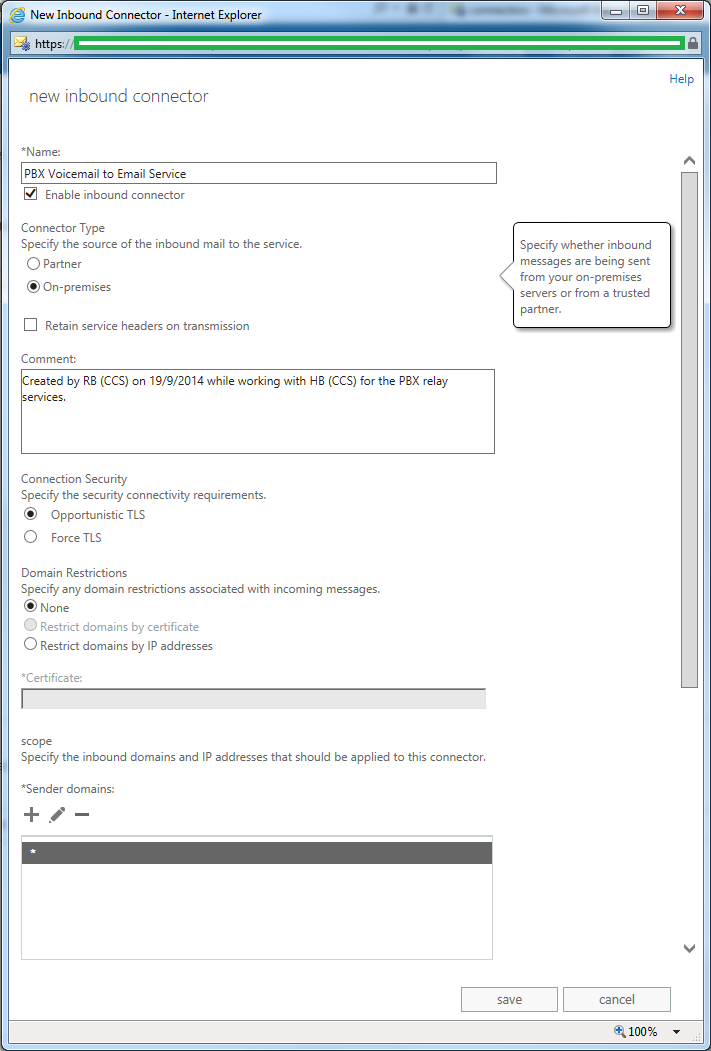The image is a screenshot of a computer screen displaying an Internet Explorer window with the title "New Inbound Connector." In the top left corner, the Internet Explorer icon, a blue lowercase "e" with a yellow swoosh, is prominently visible. Adjacent to it on the right, there are three control buttons: a minimize button, a maximize/restore button, and a close button featuring a white "X" on a red background.

Below the title, there is a green address bar where the URL would typically be entered (e.g., HTTPS). Further down, the interface includes a section labeled "Name" with a text entry field. An option labeled "Enable Inbound Connector" is present, with a check box that is marked.

The next part of the screen shows the section "Connector Type" with a description that reads, "Specify the source of the inbound mail to the service." Users can select either "Partner" or "On-premises."

Additionally, there is an option to "Retain service headers on transmission," followed by a comment box. The comment reads: "Created by RBCCS on 19-9-2014 while working with HBCCS for the PBX relay services."

At the bottom of the screen, the section titled "Connection Security" offers choices labeled "Opportunities" and "Force TLS" for configuring the security settings.